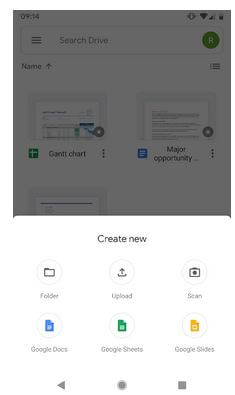Caption:  
A detailed screenshot from a smartphone taken at 9:14 AM shows the Google Drive interface. The top portion of the image is slightly grayed out but remains legible. The phone display indicates three signal bars, Wi-Fi connectivity, and a half-charged battery. An option to search within Drive and a context menu are visible at the top, alongside a green "R" icon on the far right. The main section of the screen highlights a document titled "Major Opportunity" next to an item labeled "G... Chart." Below, a white menu offers options to create new files, including folders, uploads, Google Docs, Google Sheets, and Google Slides. Additionally, the navigation bar at the bottom shows the back, home, and menu buttons typical of Android devices. This setup suggests the user is contemplating their next step within Google Drive, considering the creation of new folders or documents.